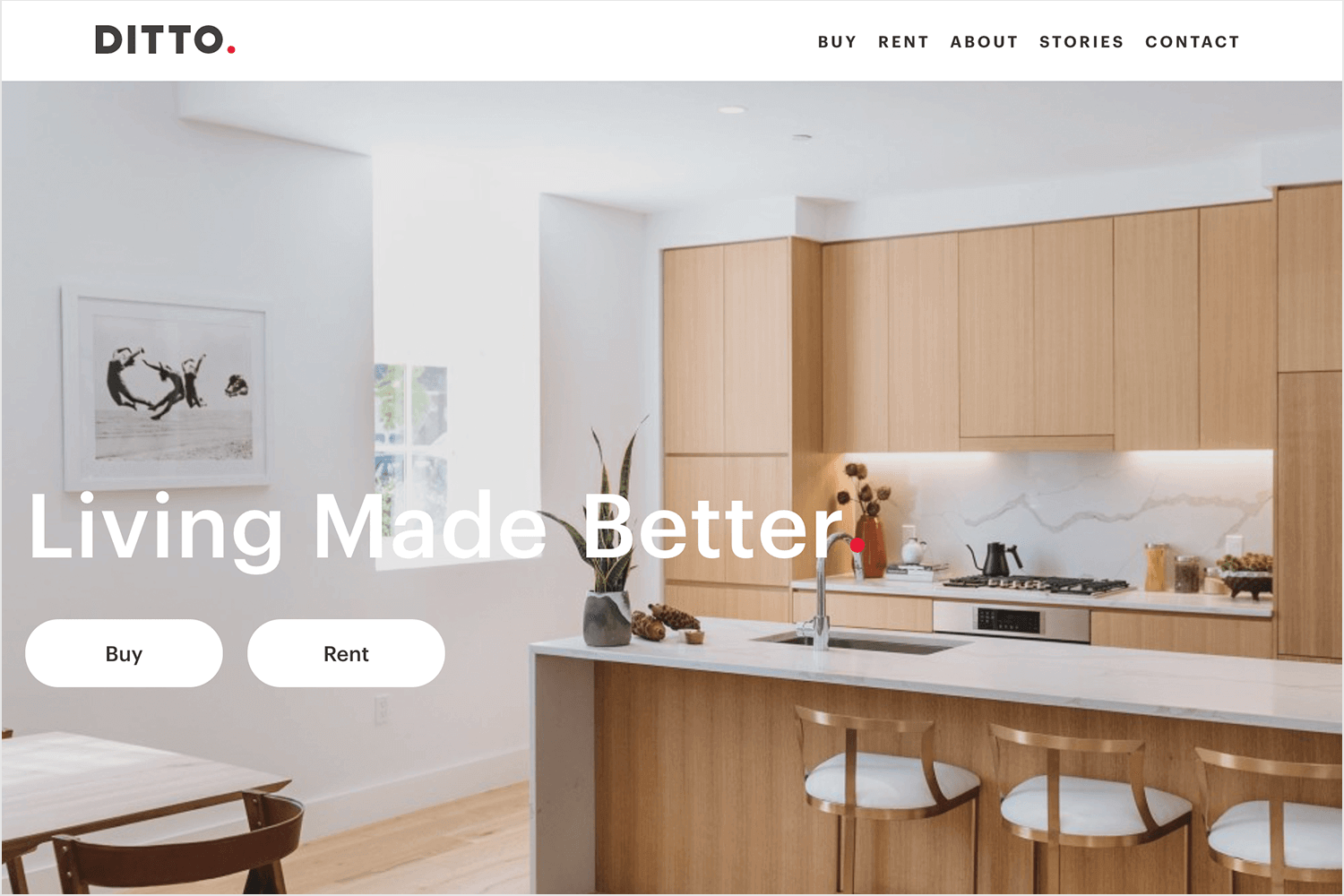A bright, welcoming kitchen is captured in this image. The centerpiece of the room is a sleek white countertop, surrounded by light brown cabinets that offer ample storage space. On the pristine white walls, a framed picture adds a touch of personality and warmth. Three chairs are neatly arranged around a sturdy table, inviting you to sit and enjoy a meal. Adding a natural touch, a few plants are strategically placed, enhancing the kitchen's serene atmosphere. At the top of the image, the words "BUY" and "RENT" are prominently displayed within black ovals, alongside options for "ABOUT," "STORIES," and "CONTACT." The word "DITTO" is boldly featured in all capitals, followed by a distinctive red dot, creating a memorable visual identity for the space.